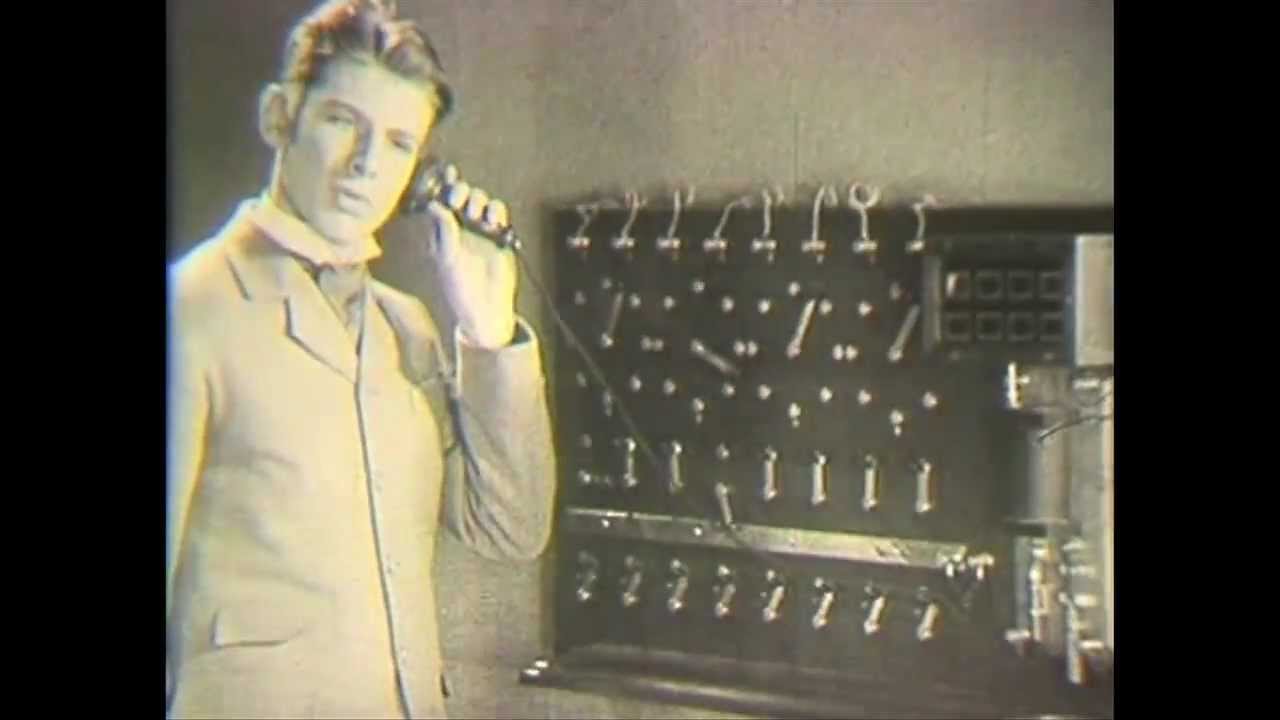This is an old black and white photograph featuring a man in his mid to late 30s, dressed in a light-colored suit with a well-groomed, slightly long black hair and a distinctive cravat or scarf under his jacket. He stands to the left side of the image, holding an old-fashioned earpiece to his left ear with a look of intense concentration on his face. The earpiece is connected to a vintage switchboard, characterized by numerous cords and switches, all set against a gray-colored wall. The photograph has a slightly grayed out or sepia tone, adding to its historical ambiance, possibly dating back several decades, potentially even to the 1960s. The man’s European features and the detailed switchboard equipment evoke a strong sense of a bygone era in telephony.